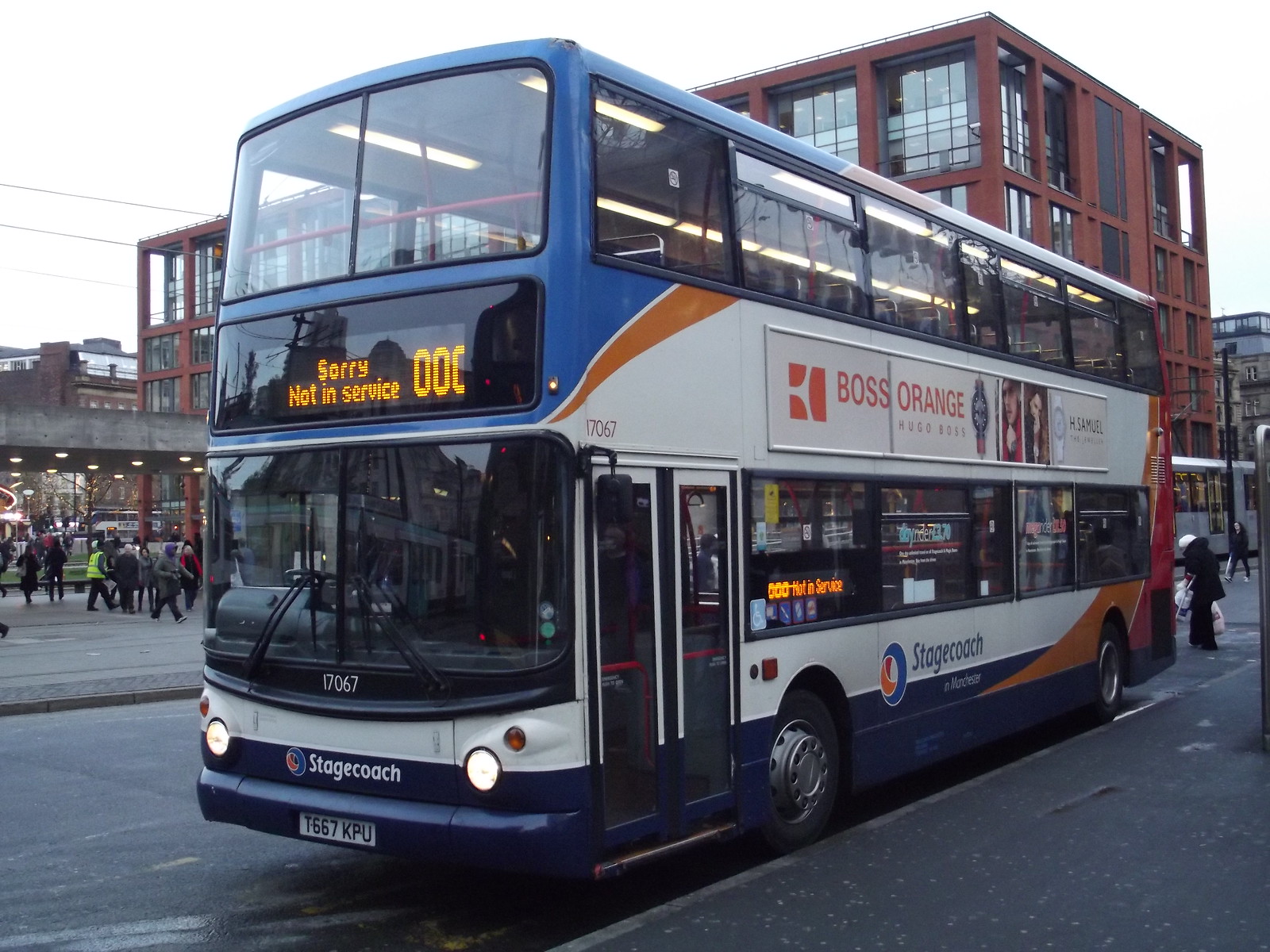In the photograph, a predominantly white double-decker bus with blue and orange stripes, and a dark blue bottom is parked centrally along a city asphalt road next to a stone sidewalk on the left. This street setting appears to be downtown, bustling with several pedestrians. The front digital sign of the bus reads, “Sorry, Not in Service, Stagecoach,” with the license plate T667KPU displayed below. The bus features an advertisement between its first and second-floor windows for "Boss Orange, Hugo Boss," showcasing wristwatch product photos. The bus has its lights on inside but no visible passengers or driver due to reflections. A multi-story brown brick building looms in the background, and additional buses suggest this might be a bus depot or major hub. Power lines crisscross against the sky at the top of the image, adding to the urban atmosphere.